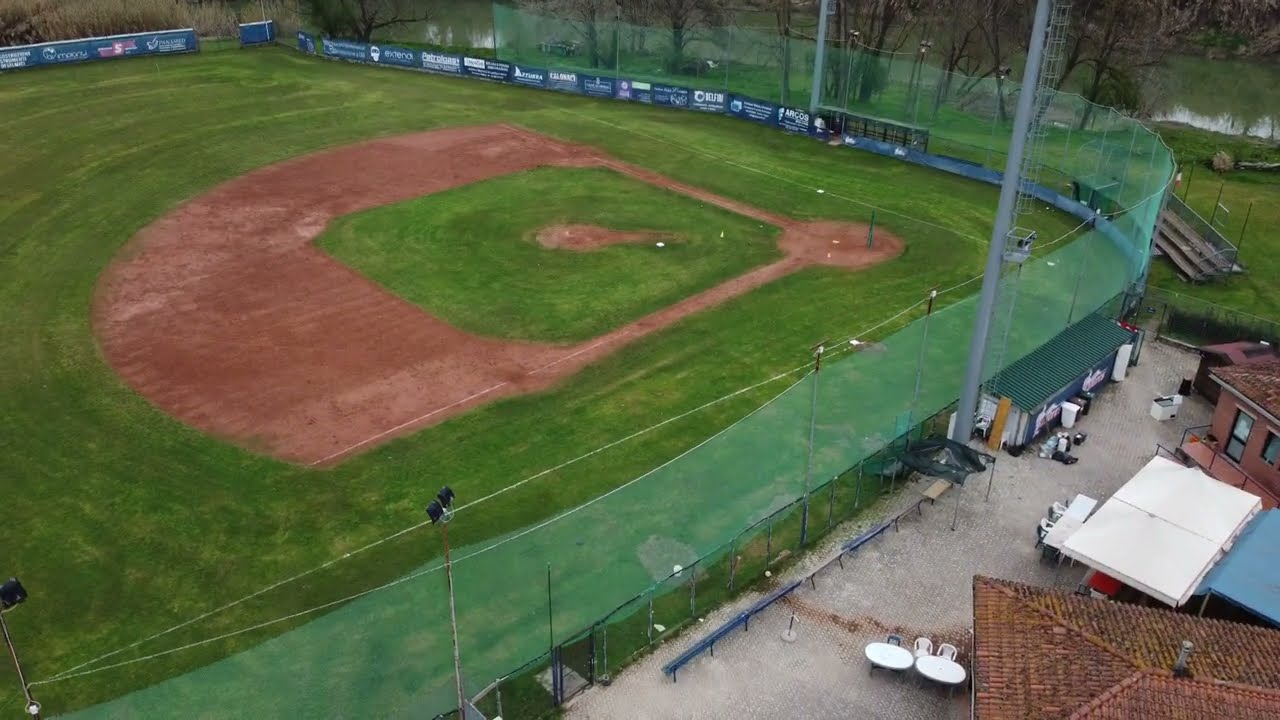This aerial, angled drone shot captures a pristine baseball field encircled by green fencing, with the drone appearing to hover about 20 feet high. The field's meticulously mowed, lush green grass, and polished brown dirt highlight its well-maintained condition. Surrounding the field are blue benches set on dirty stone tiles, and lights adorning the fence. On the image's right side, we see rooftops of small buildings, possibly cafeterias or shops, with a couple of small white tables. The bleachers are positioned in the upper right corner, adjacent to a small body of water with several skinny, hunched-over trees. Additionally, the far side of the fence is lined with numerous blue and white advertisements.